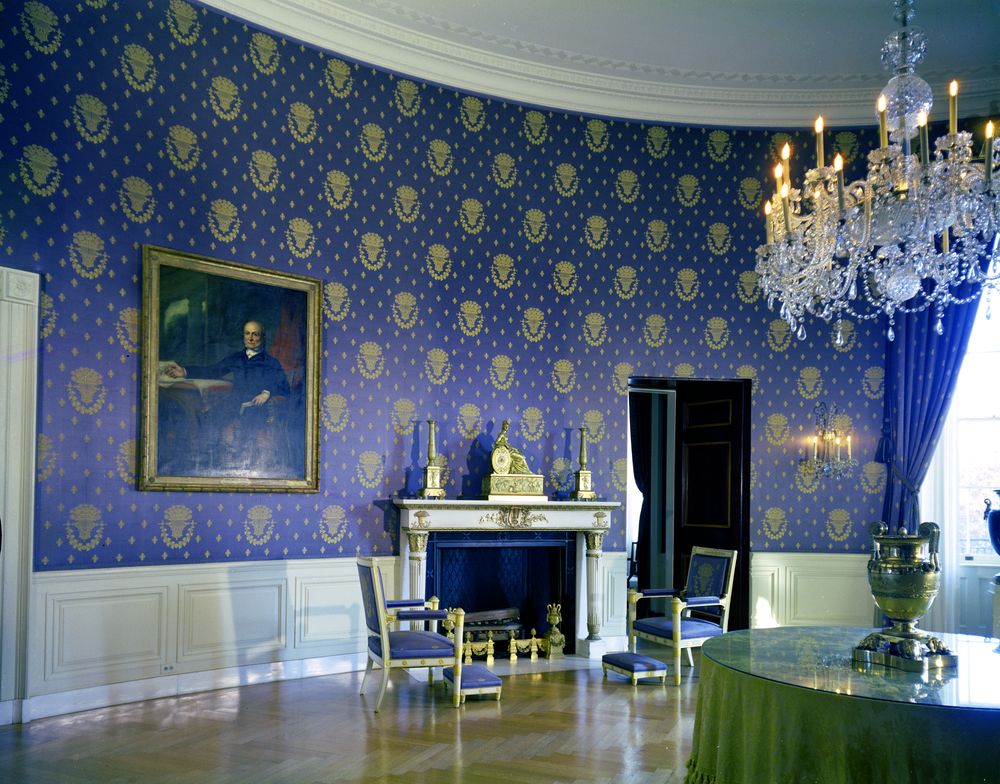The image depicts the interior of an opulent, circular room reminiscent of a royal palace or significant political building. The room is adorned with rich blue wallpaper intricately patterned with golden crests that resemble Mayan heads with wreaths underneath. A single portrait hangs on the left side of the room, portraying an elderly gentleman in a blue coat with a black collar, exuding an air of importance.

On the right side, a grand crystal chandelier with glowing flame-shaped lights illuminates the space from above. Below the chandelier, a round dining table draped in green cloth and topped with a glass cover, features an ornamental urn as its centerpiece.

The room also houses a stately marble fireplace on the lower right, framed by two chairs and matching footstools, providing a cozy yet regal touch. The mantel of the fireplace is decorated with two cantilopers and an ornate clock, enhancing the luxurious ambiance of the space. Overall, the detailed ornamentation and elegant furnishings underscore the room's majestic and historic significance.